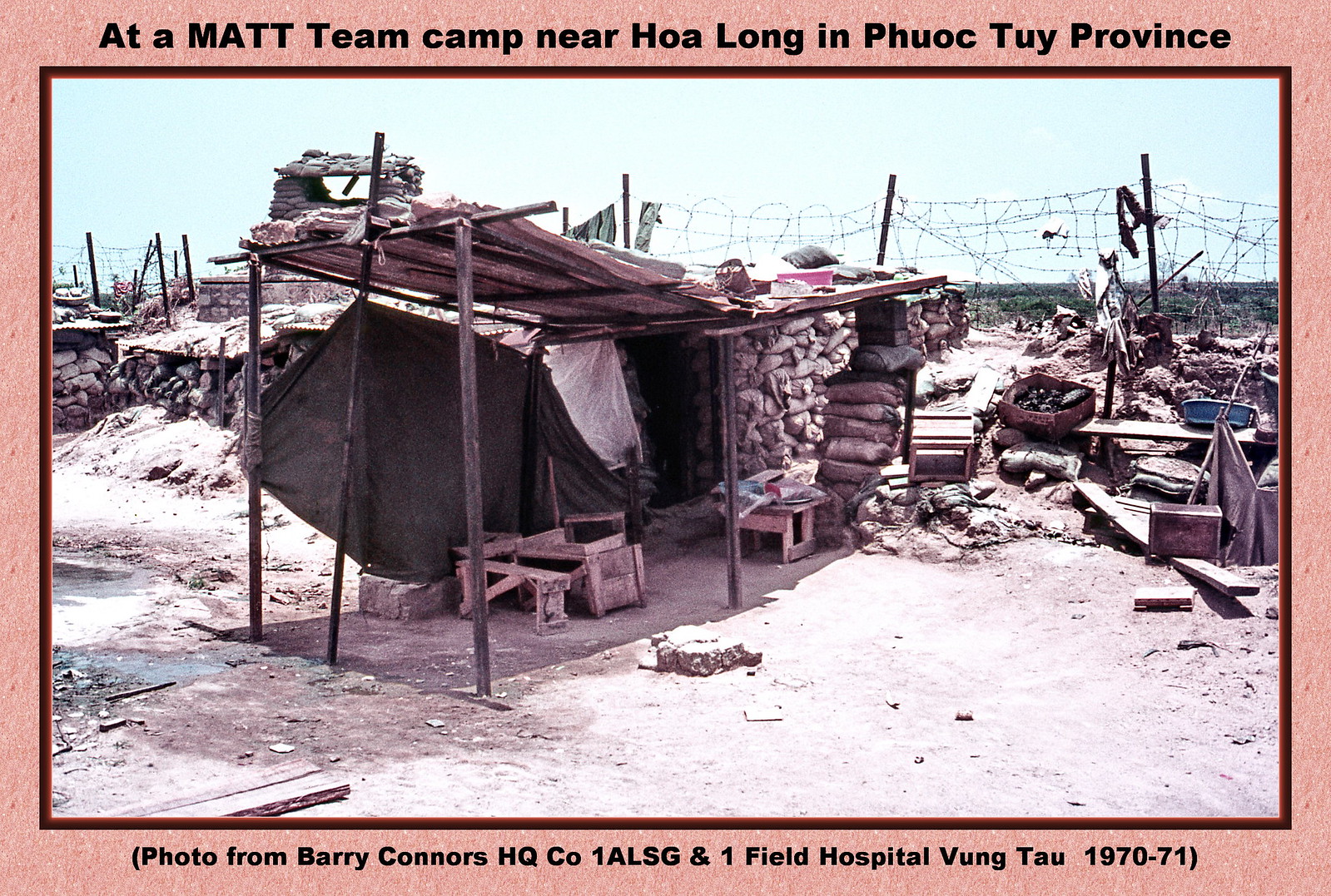The image depicts a makeshift bunker at a MATT team camp near Hoa Long in Phuoc Toi province. The photo, framed with a light red border, features black text at the top and bottom. The top label reads, "At a MATT team camp near Hoa Long in Phuoc Toi province," while the bottom label states, "Photo from Barry Connors, HQ Co. 1 ALSG and 1 Field Hospital, Vung Tau, 1970-71."

The scene shows a dilapidated shelter primarily constructed from sandbags and wooden poles, with tarps and fabric serving as the roof. The structure appears to be caving in, surrounded by wooden debris, crates, and plastic buckets scattered on the dirt ground. A shabby barbed wire fence with a visible hole runs behind the bunker, and there are patches of greenery in the far background. The faint blue sky can be seen above, but no people are present in the image.